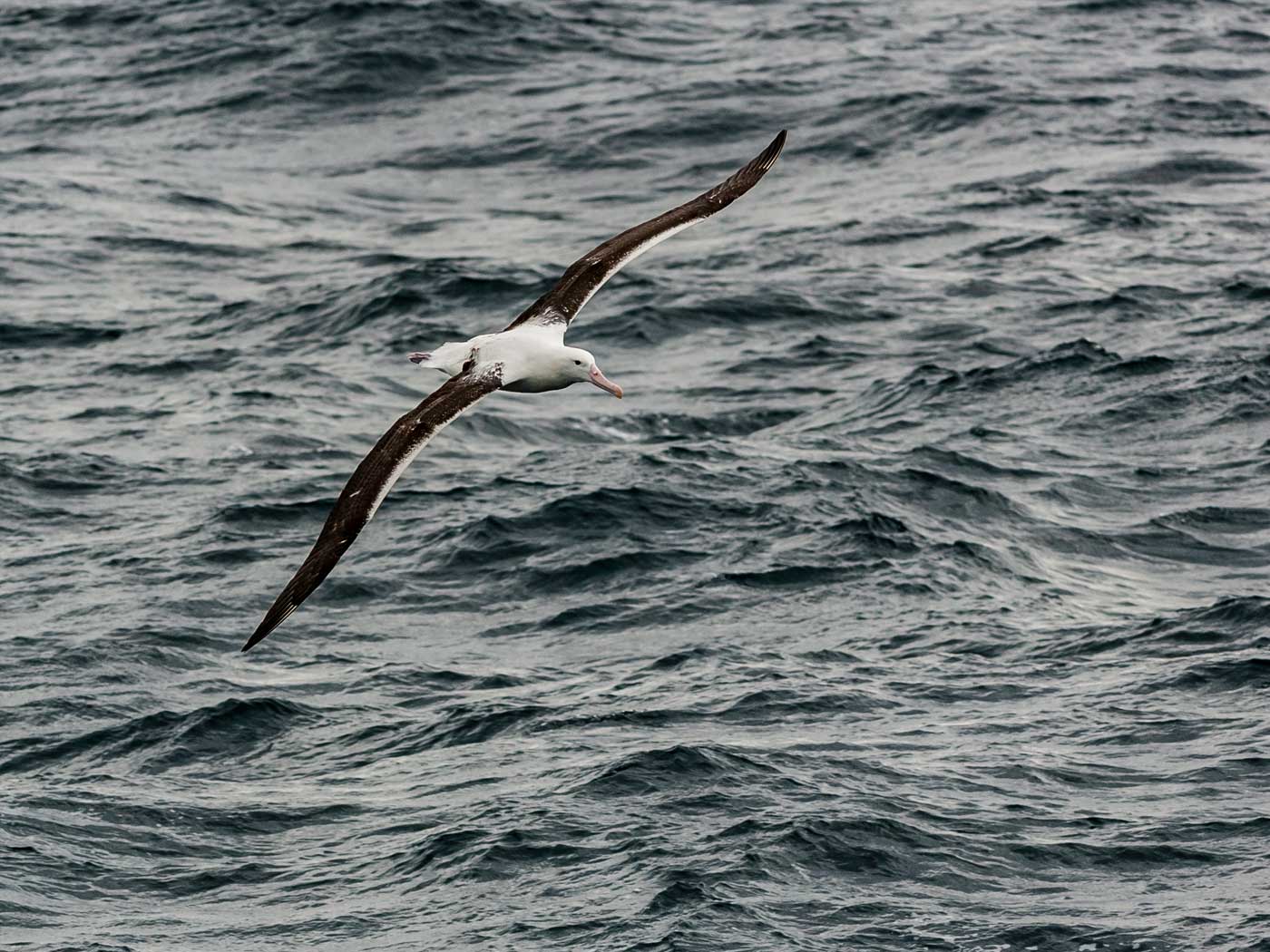In this captivating outdoor photograph, a solitary seagull with a pristine white body and strikingly long brown wings is captured in mid-flight, gliding diagonally over the swirling, choppy waves. The bird's concentrated expression is highlighted by its vivid orange, almost creamy peach beak, and piercing black eyes, suggesting a keen focus on its path ahead. Below, the open water displays a dynamic blend of colors from grayish-blue to silvery gray, with dark blue caps cresting the waves. The water’s churned and swirling appearance indicates the presence of strong winds, painting a vivid scene of nature’s raw and untamed beauty.